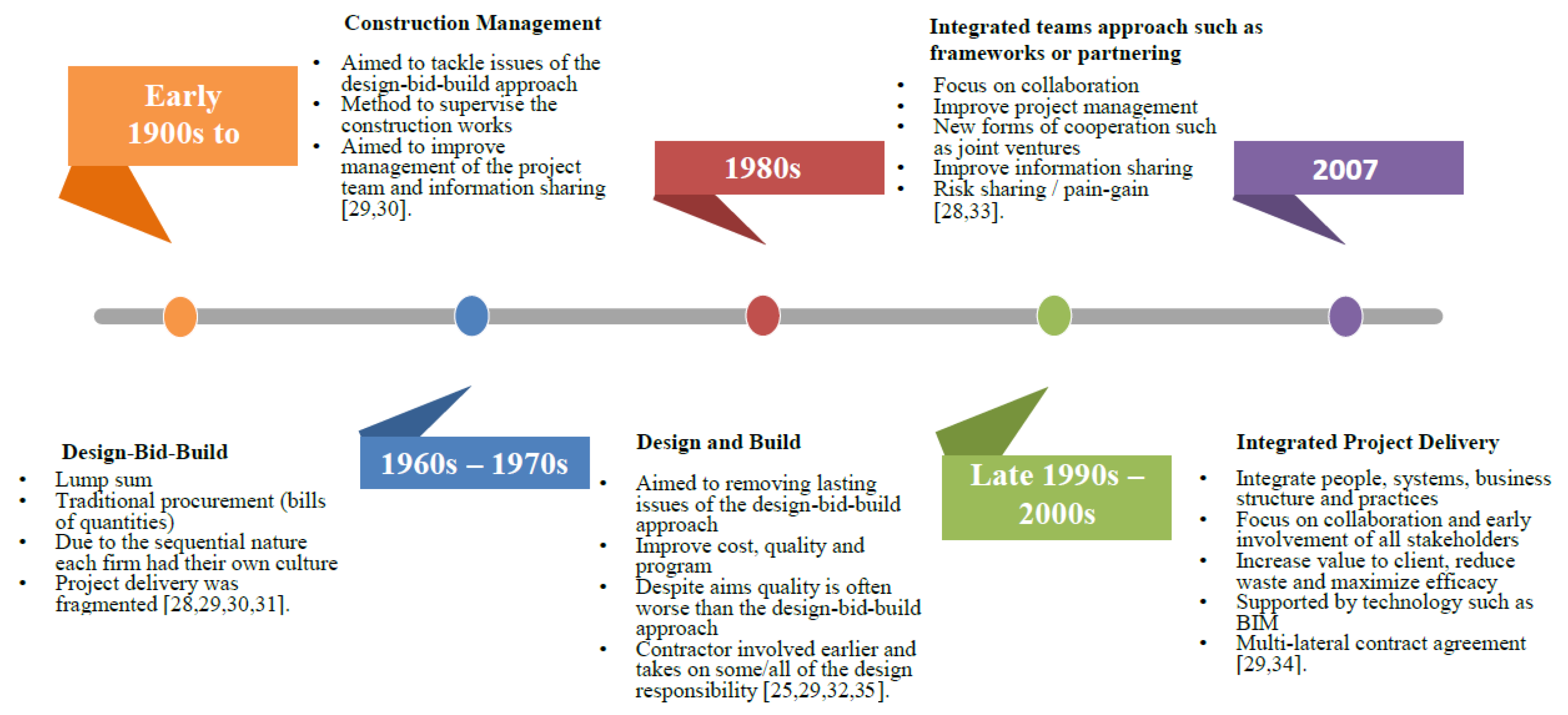The image is a detailed timeline chart on a plain white background, approximately six inches wide and three inches high, tracking the evolution of project delivery methods from the early 1900s to 2007. In the center, a horizontal gray bar with five colored circles marks significant eras. Each circle is color-coded and accompanied by banners and paragraphs of text explaining the progression.

- **Early 1900s (Orange Circle)**: An orange banner above reads "Early 1900s II." Below, black text lists "Design, Bid, Build" with bullet points: Lump Sum, Traditional Procurement, and Bills of Quantities. It notes that each firm had their own culture due to the sequential nature of projects, leading to fragmented project delivery.

- **1960s to 70s (Blue Circle)**: A blue banner below states "1960s to 70s" with "Construction Management" above. Detailed descriptions below elaborate on the construction management practices of this period.

- **1980s (Red Circle)**: A red banner above mentions "1980s" with "Design and Build" beneath. The text elaborates on this integrated approach.

- **Late 1990s to Early 2000s (Green Circle)**: A green banner below indicates "Late 1990s to 2000s." Above, it states "Integrated Teams Approach," discussing frameworks or partnering as key strategies of this era.

- **2007 (Purple Circle)**: A purple banner above reads "2007." Below, "Integrated Project Delivery" is explained, emphasizing collaboration and efficiency.

The chart collectively highlights the evolution of project delivery methods, showing a progression from traditional, fragmented approaches to more integrated and collaborative methods.